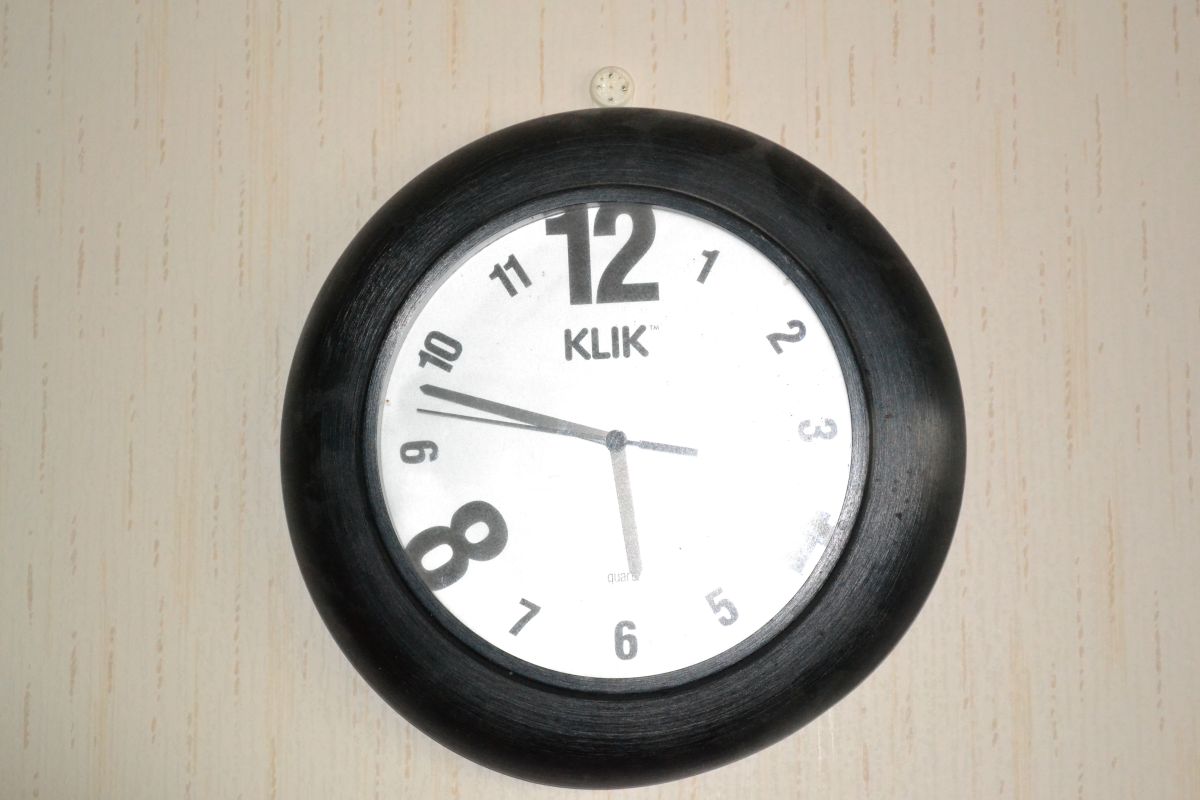This photograph showcases a circular, black-framed wall clock with a white face and black hands for the seconds, minutes, and hours. The clock prominently features an unusually large number 12 and number 8, which are significantly larger than the rest of the numerals. Despite the missing number 4, all other numbers are present and uniformly sized. The clock face is glossy, suggesting the use of a flash in capturing the image, and the current time is 5:48, or 12 minutes to 6. The brand name "KLIK" is also visible. The clock is mounted on a wall that resembles light wood paneling or possibly wood-grain wallpaper.